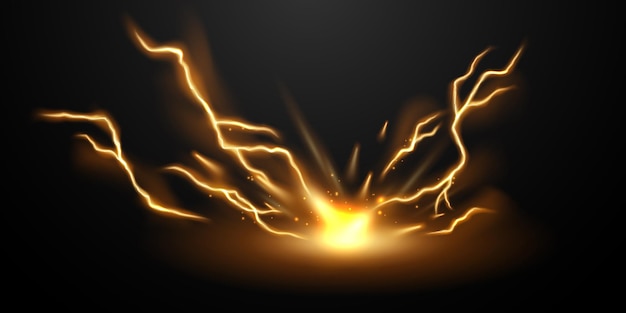The image appears to be a computer-generated depiction of a central bright, glowing object emitting streaks of light against a predominantly black background. The focal point in the middle consists of a bright yellow, white, and orange light that resembles a flame or an eruption. From this central glow, jagged and crooked lines extend outward, mimicking the appearance of lightning or tree branches. These streaks of light shoot off in various directions, with some detached and others connected, creating a dynamic scene. The background is black, fading into brown near the light source, and is dotted with small orange specks resembling embers or sparks emanating from the central light. The overall effect conveys a vivid and energetic display of light, shadow, and color.